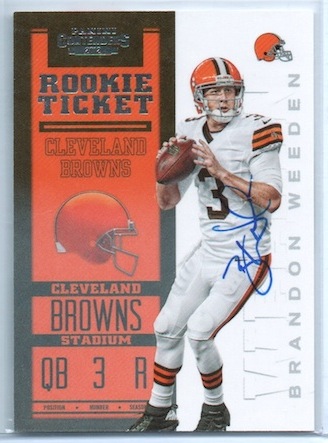The image is a color photograph of a football trading card, specifically a rookie card, styled similarly to a classic baseball card. The card is in portrait orientation, with a Cleveland Browns player, Brandon Weeden, prominently featured on the right side. He is pictured holding a football in a posed, active stance, seemingly preparing to throw it. Weeden is wearing a white uniform with orange and brown stripes and a matching helmet. His number, 3, is clearly visible on his chest, and his name, "Brandon Weeden," is written vertically along the right-hand side of the card in a gray font.

The left side of the card is dominated by an orange rectangle containing various pieces of text and information. At the top, it reads "Rookie Ticket" followed by "Cleveland Browns," beneath which is an orange Browns helmet. Further down, the words "Cleveland Browns Stadium" are written, with his rookie designation "QB 3R" indicating his quarterback position. The card also features Weeden's blue signature. This card exemplifies photographic realism, capturing the player in authentic detail.